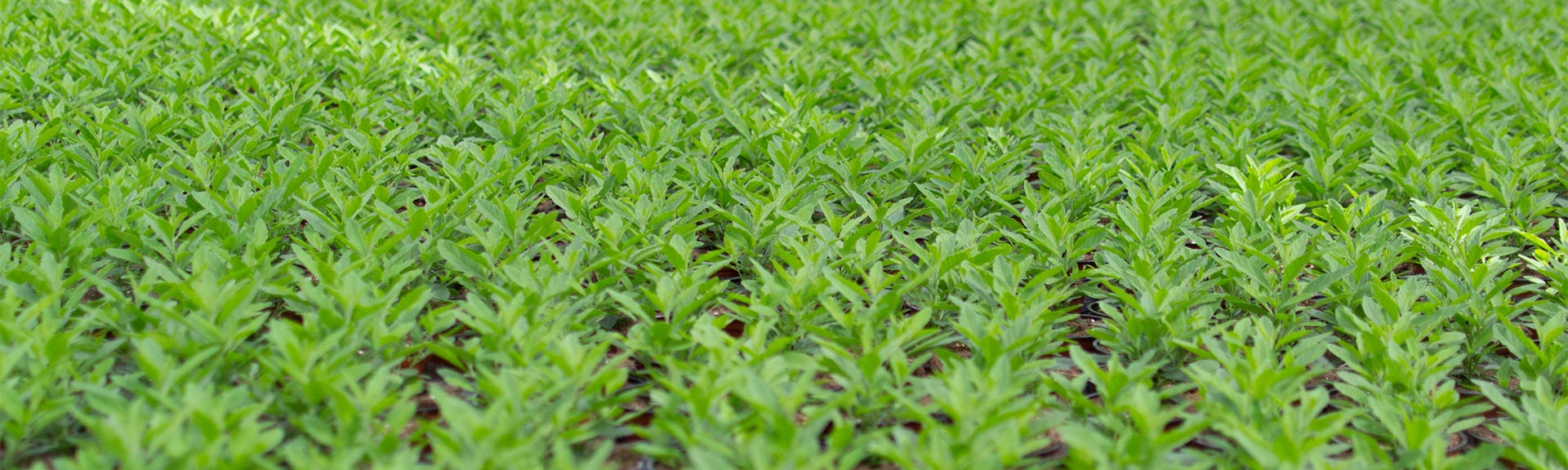This photograph captures a vibrant field of small green plants with several budding leaves, neatly arranged in approximately 20 uniform rows, each containing around 10 to 20 plants. These plants, which appear to be of the same variety, are uniformly green and similar in height, giving the field a very tidy and consistent look. Between the rows, patches of brown soil are visible, hinting at careful cultivation.

A significant feature of the image is a ray of sunlight, which streams diagonally from the top left corner to the middle right, intermittently illuminating the green leaves. This light creates subtle variations in the green hues, ranging from a rich, deep green to a lighter shade, enhancing the lush and healthy appearance of the plants. The entire photograph, taken from a close-up perspective, emphasizes the dense, orderly planting, with no other objects in sight, just the thriving plants and the soil they sprout from. The image has a wide format, about four times wider than it is tall, capturing the expanse of this well-maintained field.